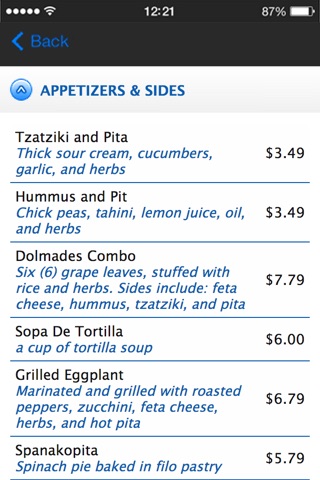This image is a screenshot of a digital menu, prominently displaying details about appetizers and side dishes. At the top of the screen, there are standard icons including a wireless signal indicator, network strength bars, the current time, and battery percentage. A blue back button is located at the upper left corner of the menu interface. 

The menu section titled "Appetizers and Side Dishes" lists a variety of food items with detailed descriptions and prices:

1. **Tzatziki and Pita** - A dish featuring thick sour cream, cucumbers, garlic, and herbs, priced at $3.49.
2. **Hummus and Pita** - A combination of chickpeas, tahini, lemon juice, oil, and herbs, available for $3.49.
3. **Dolmathes Combo** - Includes six grape leaves stuffed with rice and herbs, accompanied by sides such as feta cheese, hummus, tzatziki, and pita, priced at $7.79.
4. **Sopa de Tortilla** - A cup of tortilla soup, offered for $6.00.
5. **Grilled Eggplant** - Marinated and grilled eggplant served with roasted peppers, zucchini, feta cheese, herbs, and hot pita, priced at $6.79.
6. **Spanakopita** - A spinach pie baked in phyllo pastry, available for $5.79.

The background of the menu is predominantly white, with the menu title in black and the ingredients or side details highlighted in blue text.